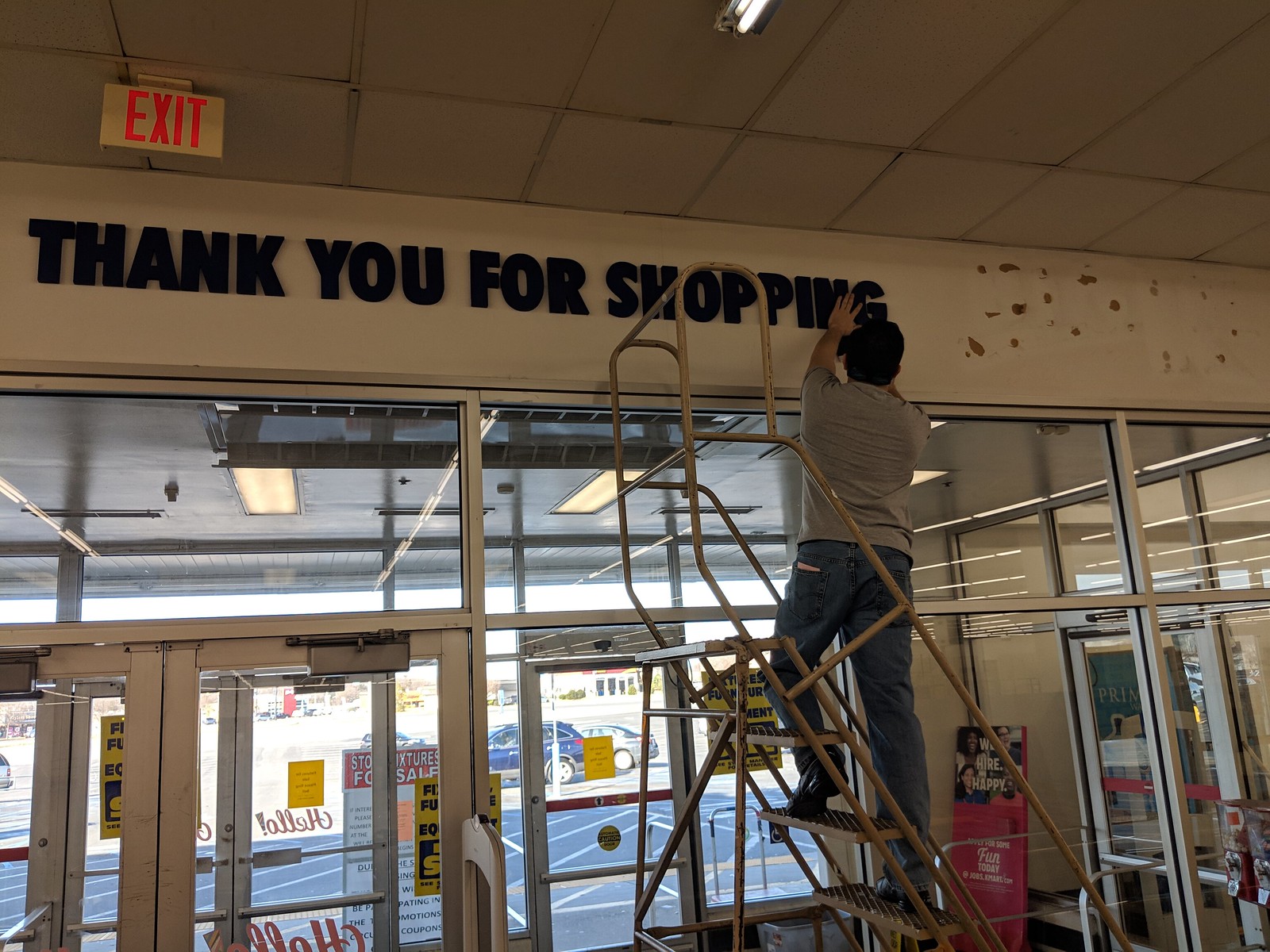In front of a store's exit, a sign mounted on the ceiling glows with neon red letters spelling out "EXIT." A man dressed in a gray short-sleeved shirt and jeans is working atop a silvery ladder, affixing black letters that read "Thank you for shopping" above the white automatic doors. The doors themselves are adorned with red and white font and display a hiring sign that says "We hire happy" in white text. Above the doors, glass panels capture reflections of lights, while some of the doors feature black and yellow signs. Beyond the entrance, a partial view of the parking lot reveals a silver car and a bluish car parked in the background, with the exterior lights reflecting off the surrounding glass.